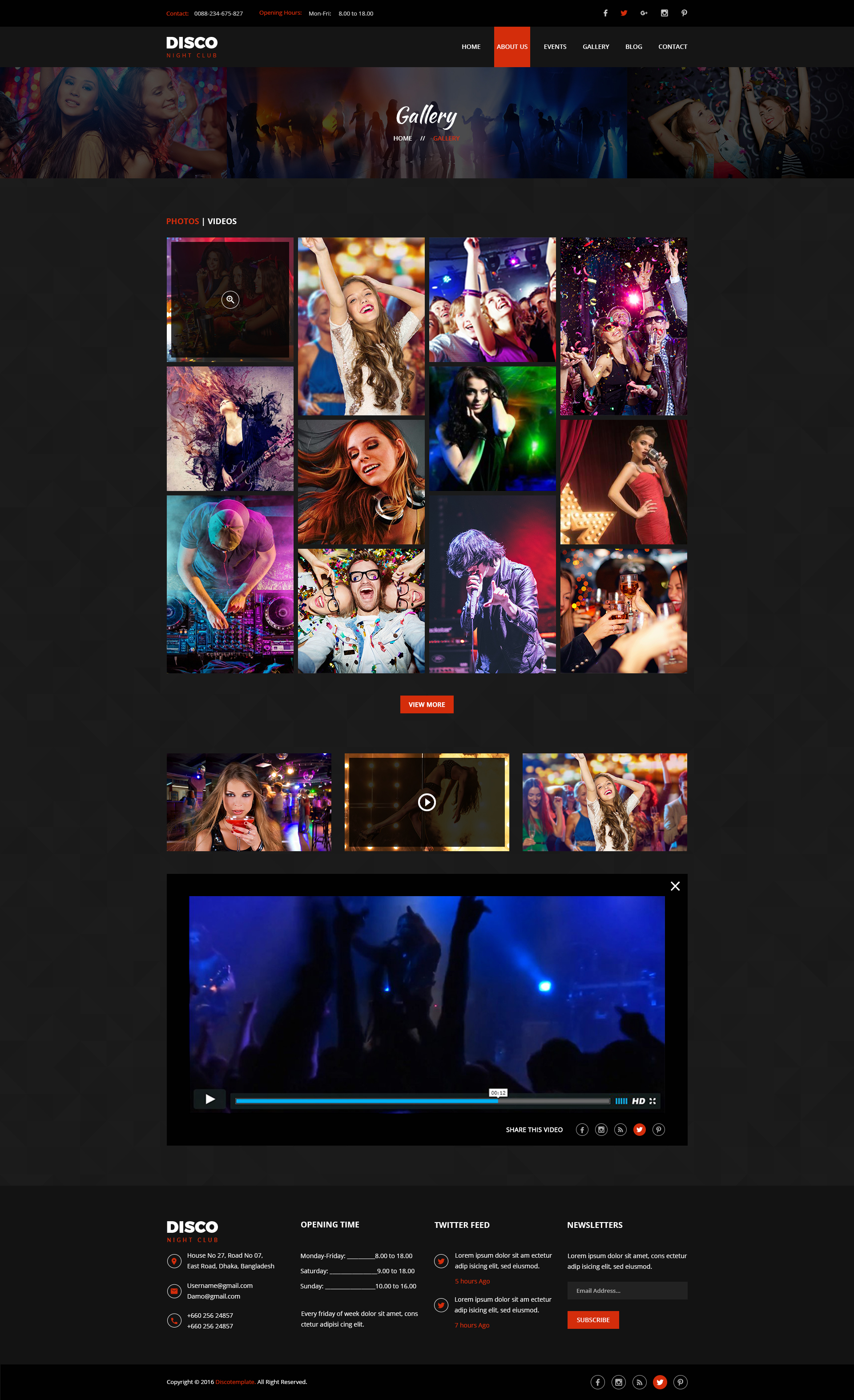The website features a predominantly light black background with a sleek, modern aesthetic. At the top left corner, the main title of the website reads "Disco" in bold white text, with the tagline "An Orange Nightclub" displayed just underneath in vibrant orange. The header of the webpage includes a solid black navigation bar running across the top, containing some partially legible orange and white text on the left side. 

Embedded within this top section, the top right corner showcases icons for prominent social media platforms, including Facebook, Twitter, and Google. Positioned to the right of the "Disco" text, there is a navigation menu with six options written in white: Home, About Us, Events, Gallery, Blog, and Contact. The "About Us" option stands out, highlighted in bright orange.

Directly beneath the navigation menu is a wide banner with the word "Gallery" prominently displayed in white text at its center. Below the banner, there are three distinct images: the central image portrays a lively dance floor filled with silhouettes in motion, the left image captures two girls standing back to back with their hair flowing, and the right image features two girls with raised arms, beaming with smiles.

In the middle section of the website, there is a structured square layout showcasing four columns of photographs, with each column containing three images of varying sizes. The photos depict people enjoying themselves—smiling, singing, and dancing against a backdrop of vibrant nightlife scenes. Just below this photo gallery is a striking red button that reads "View More" in bold white text.

Further down, there is a video player embedded into the page, indicating multimedia content is available. Finally, the footer of the website is rich in information. It includes sections labeled "Disco," "Opening Times," "Twitter Feed," and "Newsletters," filled with additional details. The bottom right corner features icons for Facebook, email, and Twitter, while the bottom left corner includes a copyright notice, rounding off the page with essential contact and legal information.